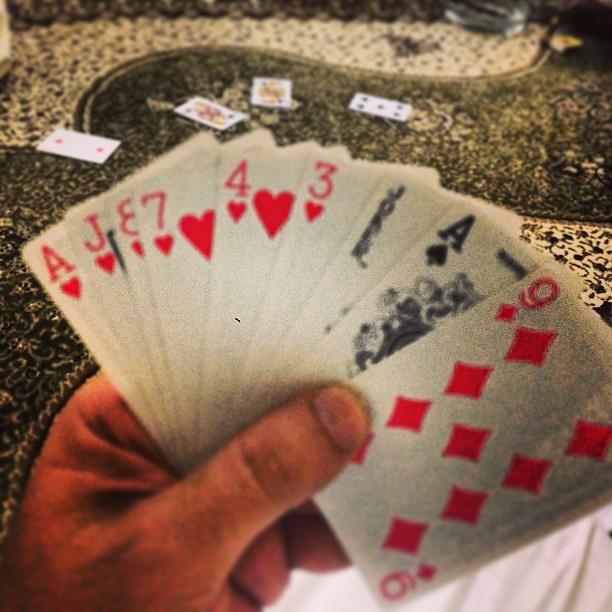The image features a close-up of a hand holding a fanned-out assortment of playing cards. The hand is prominently displayed against the backdrop of a black-and-white tiled table. The cards held include the Ace of Hearts, the Jack of Hearts, the Eight of Hearts, the Seven of Hearts, the Four of Hearts, the Three of Hearts, the Joker, the Ace of Spades, and the Nine of Diamonds. On the table behind the hand, four additional playing cards are laid face-up, consisting of three black-suited cards and one red-suited card. The scene is set at a card table, capturing the intricate details of the cards and the setting.